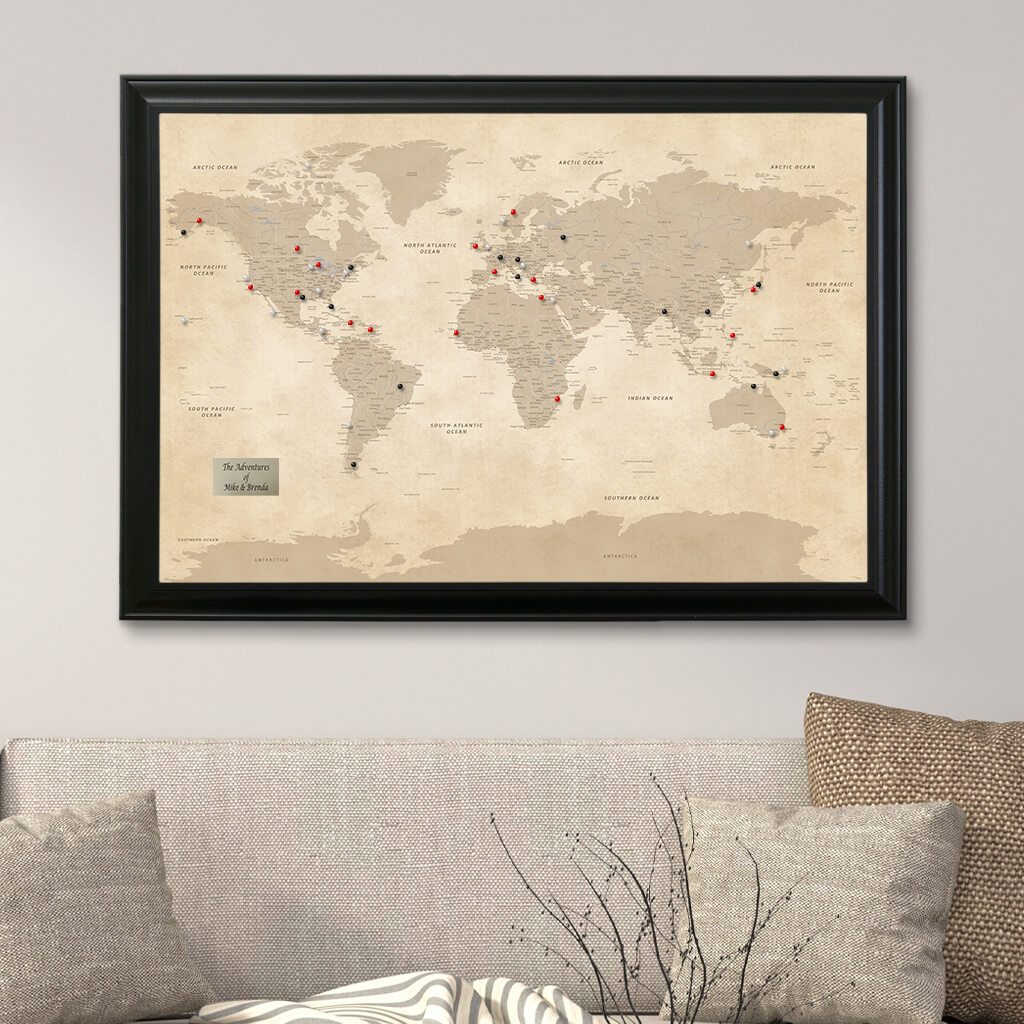In this image of a living room, the walls are painted a light gray and feature a large, black-framed world map prominently displayed above a cozy light gray couch. The map, which appears to be a globe laid out flat, showcases all the continents and is dotted with red and black stick pins, potentially marking destinations the resident has visited or wishes to explore. The couch, positioned in the forefront, is adorned with three throw pillows - two in gray that match the couch's weave, and a larger one in a tan and white pattern. Adding to the comfort and decor, a throw blanket is draped over the couch, and a vase filled with decorative sticks sits on a coffee table in front of it.